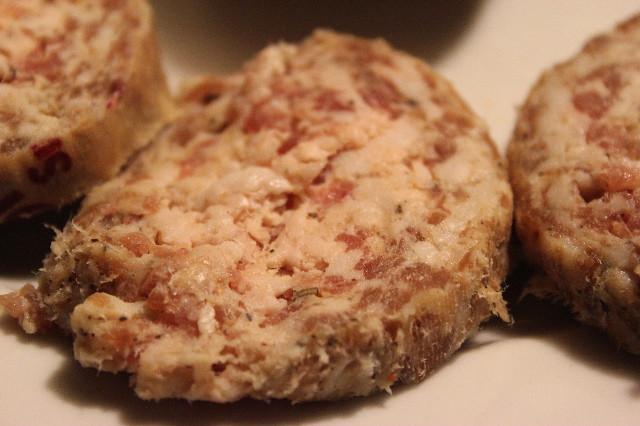This is an extreme close-up photograph of what appears to be bulk pork, potentially sausage, featuring three pieces arranged on a flat, tan-colored surface, likely a kitchen counter or a piece of meat wrapping paper. The focal point is the circular cut of meat in the center, which nearly occupies the entire frame. The center piece is a rounded, red and white marbled meat, showcasing a significant amount of fat. To the left and right, partially in and out of the frame, are two additional pieces. The leftmost piece has some labeling or print, indicating it could be encased in sausage skin. The setup suggests no people, text, or date, and the photo is taken indoors, inferred from the lighting and absence of shadows. The overall composition hints at a display or preparation of the meat pieces.